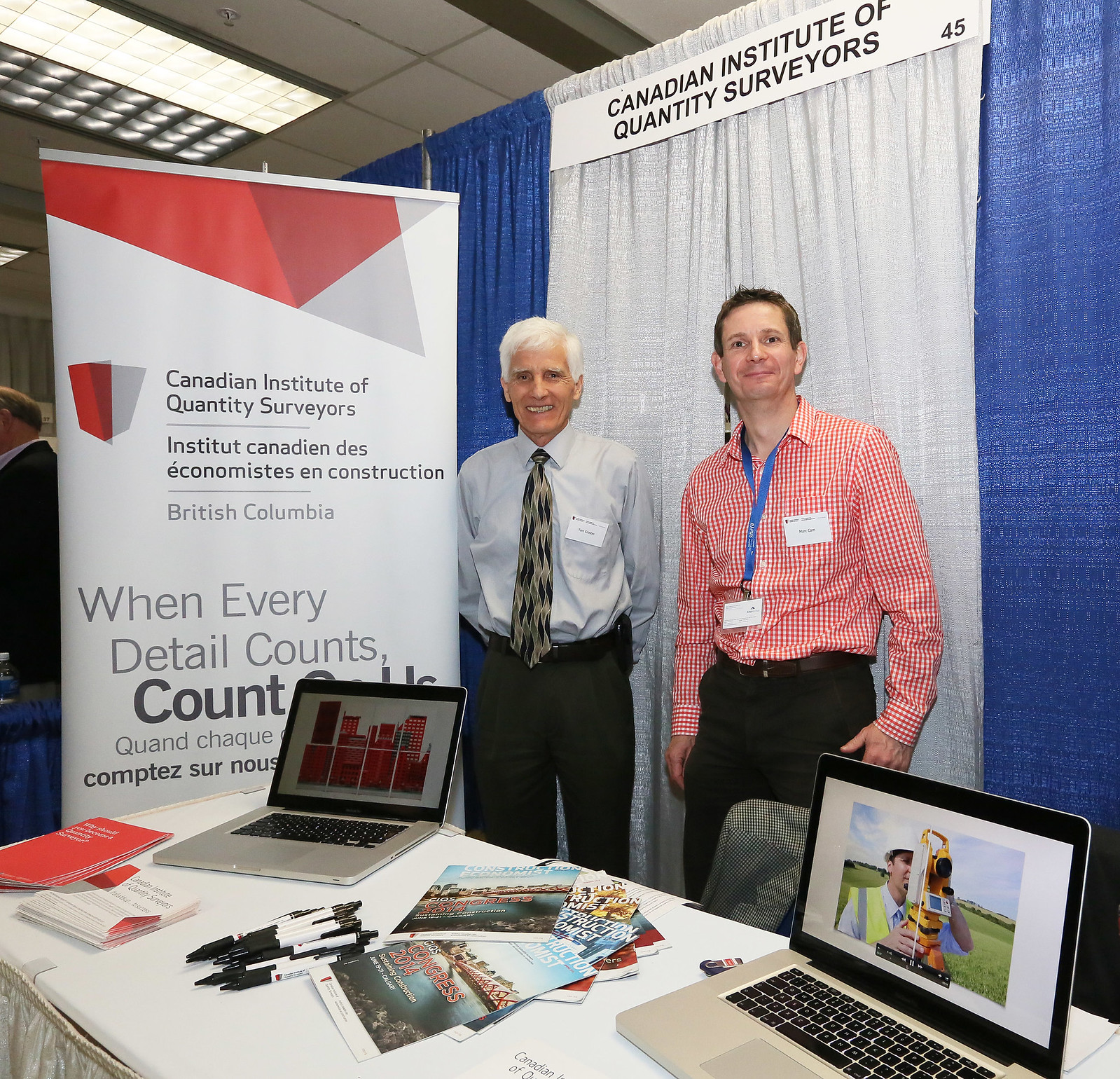In this detailed photograph, we see a booth at a business expo, specifically Booth 45, representing the Canadian Institute of Quantity Surveyors. The scene is set with a white and blue curtain as the backdrop. In front of this curtain stand two gentlemen, both seated behind a table draped with a white cloth. On the table are two open laptop computers, a collection of pens, and various reading materials pertaining to their business, emphasizing the slogan "Every detail counts. Count on us."

The gentleman on the left, appearing older with white hair, is dressed in charcoal slacks, a light blue shirt, and a gray tie. The gentleman on the right sports brown hair and wears a red and white striped collared shirt paired with brown slacks. Both men have name tags affixed to their attire. Their detailed setup and the comprehensive signage, including a banner that prominently reads "Canadian Institute of Quantity Surveyors," underscore their commitment to precision and professionalism in their field.